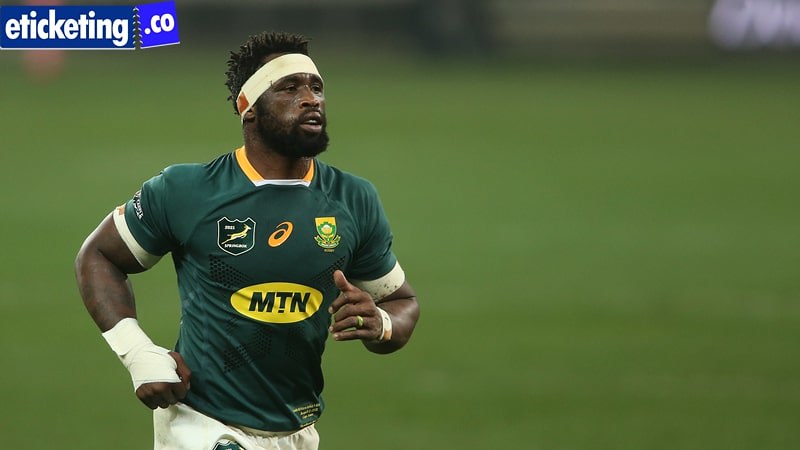The photograph captures a focused moment in a soccer game featuring a Black player in mid-action, seemingly running, with his body cut off just below the waist. He is wearing a vivid forest green short-sleeved jersey adorned with a yellow oval center emblazoned with 'MTN' and three sponsor logos above it. His crisp white shorts are partly visible. The player sports a white headband accentuating his short dreadlock-like hair, along with a black beard and mustache shaping his face. His right hand and wrist are wrapped with white tape, while his left hand is adorned with a gold ring and a bracelet. The background consists of a blurry green grass field, emphasizing the player's sharp focus. In the upper right corner, part of the image features a blurry banner with text, including ".co" and "e-ticketing."